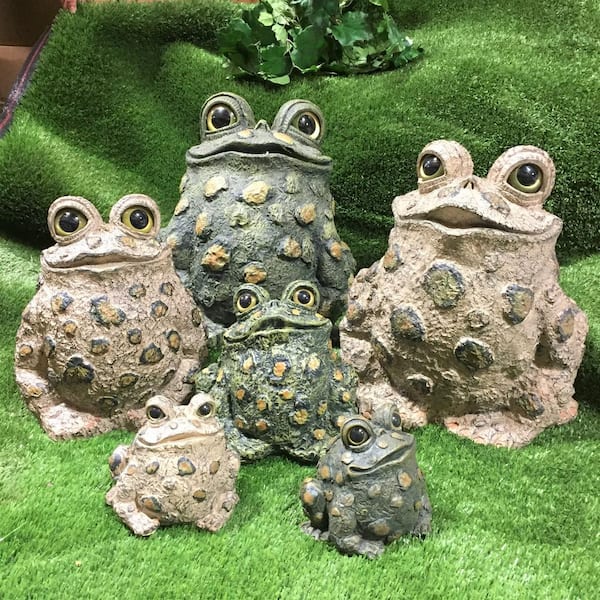The photograph features a collection of six frog and toad figurines, likely made of ceramic or clay, with a notably rough, pebbly texture. Arranged in two rows, the three larger figurines are situated in the rear while the three smaller ones reside in the front. These amphibious statuettes exhibit a mix of light gray, light brown, dark green, and dark gray colors, each adorned with contrasting circular spots or warts. They have distinct, open-mouthed smiles and prominent turreted eyes perched atop their heads. The figurines rest on a surface resembling astroturf, a short, fuzzy green material, and a hint of a wooden table is visible in the upper left-hand corner of the photo. Additionally, a small bush or shrubbery is faintly seen at the top edge of the green surface. All the figurines face the camera, except for one small green frog, which is turned to the left.